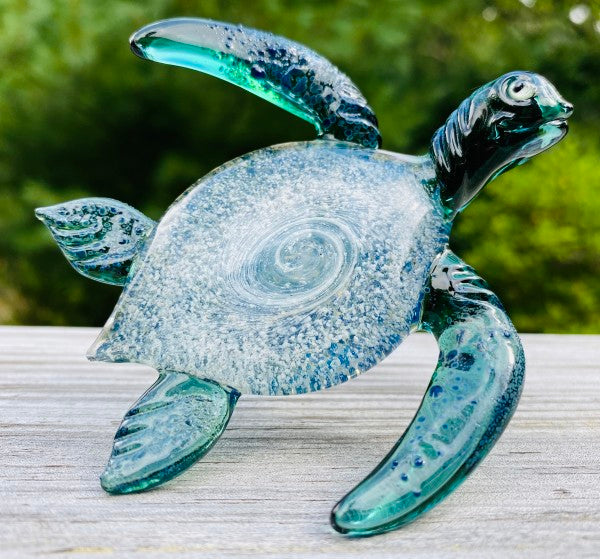The image features a meticulously crafted, turquoise glass-blown sea turtle positioned upright on a light grey and brownish wooden surface. The turtle's vibrant, bluish-green hue is accentuated with embedded bubbles and a swirling pattern of different shades of blue and white throughout its textured shell, creating a captivating visual effect. The background, captured on someone's camera phone, is intentionally blurred, emphasizing the sea turtle while hinting at lush green foliage and tree shapes, suggesting an outdoor setting. The glass turtle, poised as if in motion, presents a striking decorative piece that would look stunning in any setting, be it a desk or an entertainment unit.